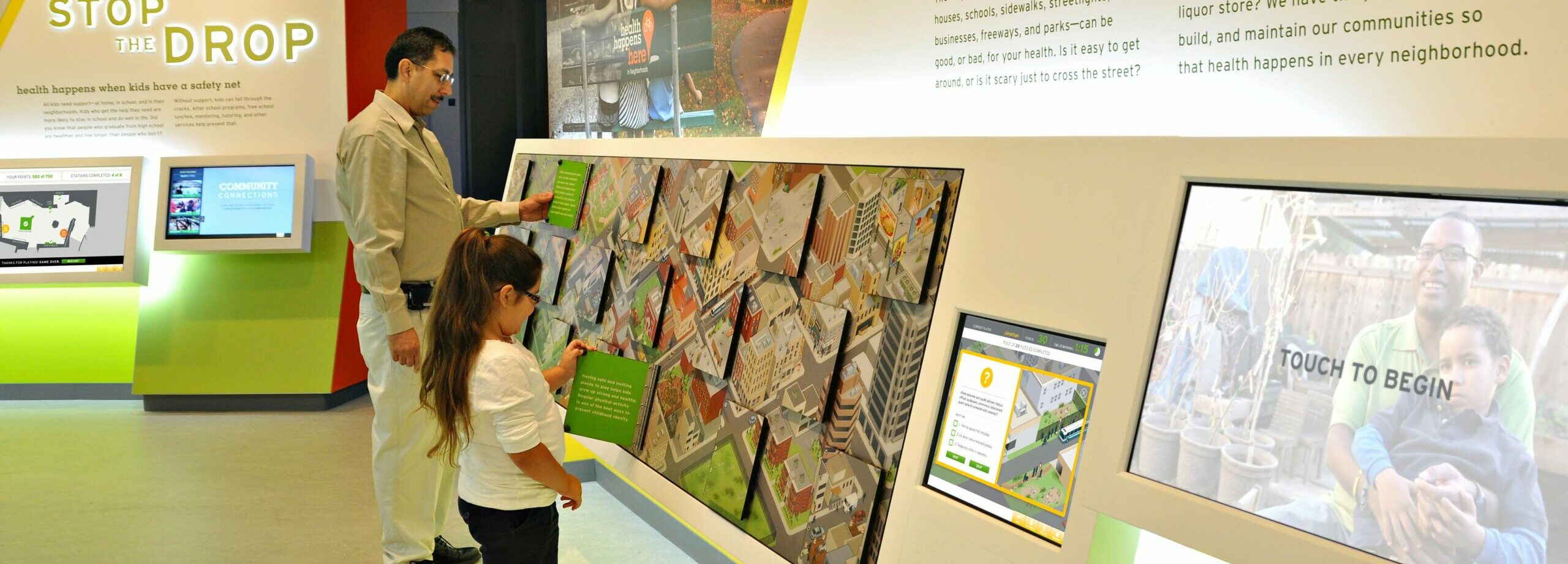The image depicts an indoor exhibition scene focused on city planning or development. Two individuals, a man and a young girl, are looking at a detailed display mounted on the bottom part of a tan-colored wall. The display showcases a planned city or area of a city, with various sections marked by small square plaques identifying residential, commercial, and green areas. Each plaque is easily readable, providing specific details about the area's characteristics.

The man on the left is wearing a beige shirt and white pants, and he appears to be intently examining the display. To his right, the young girl, dressed in a white shirt and black pants with long hair flowing down her back, is also engaged with the exhibit. In the lower right corner of the display, a computer monitor invites interaction with a "Touch to Begin" prompt. 

In the background, a larger sign reads "Stop the Drop," accompanied by the message, "Health happens when kids have a safety net." Below this sign, there are two computer screens or viewing areas providing additional information. The entire setup appears to educate viewers on the planned development and its various zones, emphasizing the importance of thoughtful city planning.